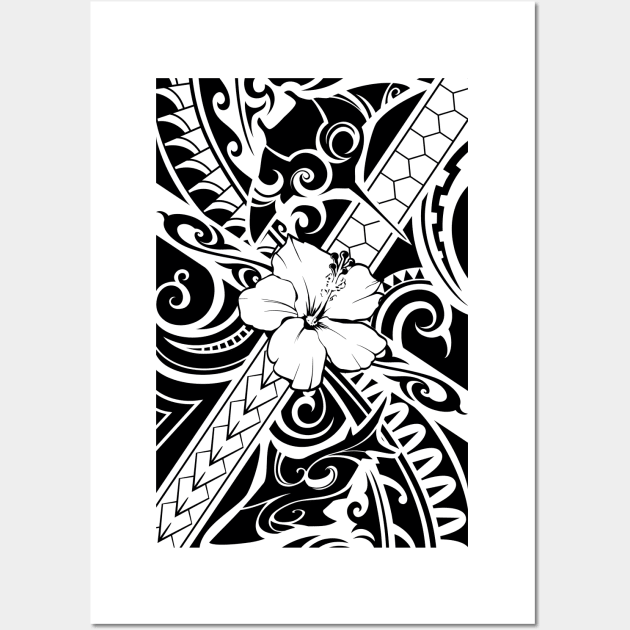This detailed black and white illustration features intricate line art set against a light gray wall. At the center of the piece, a white hibiscus flower is depicted prominently, with a large stamen and anther extending outward. Surrounding the hibiscus are a variety of geometric and organic designs, including tribal-like patterns with repeated shapes such as triangles, squares, and curves. Above the flower, a black and white manta ray with deliberate white designs is illustrated, giving it a striking appearance. Below the flower runs a band with distinctive decorative elements – on one side, a honeycomb pattern, and on the other, an arrowhead design. Additionally, there's a ribbon-like shape adorned with U-shaped designs along the band. The artwork, seemingly computer-generated with clean and precise lines, is bordered by a white frame and stands out vividly against its surrounding, though it lacks an artist's signature.